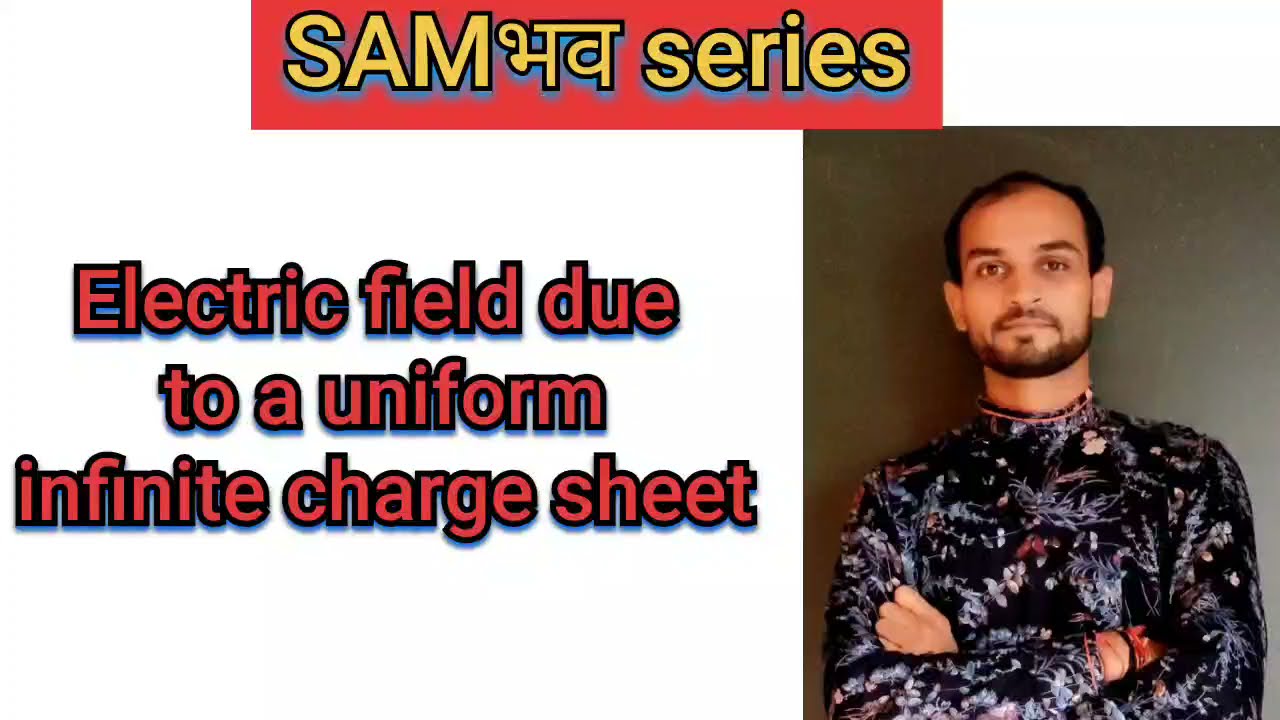The image resembles a PowerPoint slide, predominantly featuring a semi-formal photograph of a man and some informative text. Positioned on the right side of the image is a man of likely Middle Eastern or Indian descent, with slightly darker skin, short black hair, and a neatly trimmed black beard. He gazes forward with a serious expression and his arms crossed over his chest. He is attired in a dark blue shirt adorned with a vibrant floral pattern. The background behind him is a plain, neutral gray.

At the top of the image, a red rectangular text box displays the word "SAM" in capitalized yellow letters with a blue outline, followed by a series of foreign characters that appear to be Southeast Asian, possibly Arabic or another script type, and the word "series" in lowercase letters. Centered on the main part of the image, a red text with a black border reads, "electric field due to a uniform infinite charged sheet."